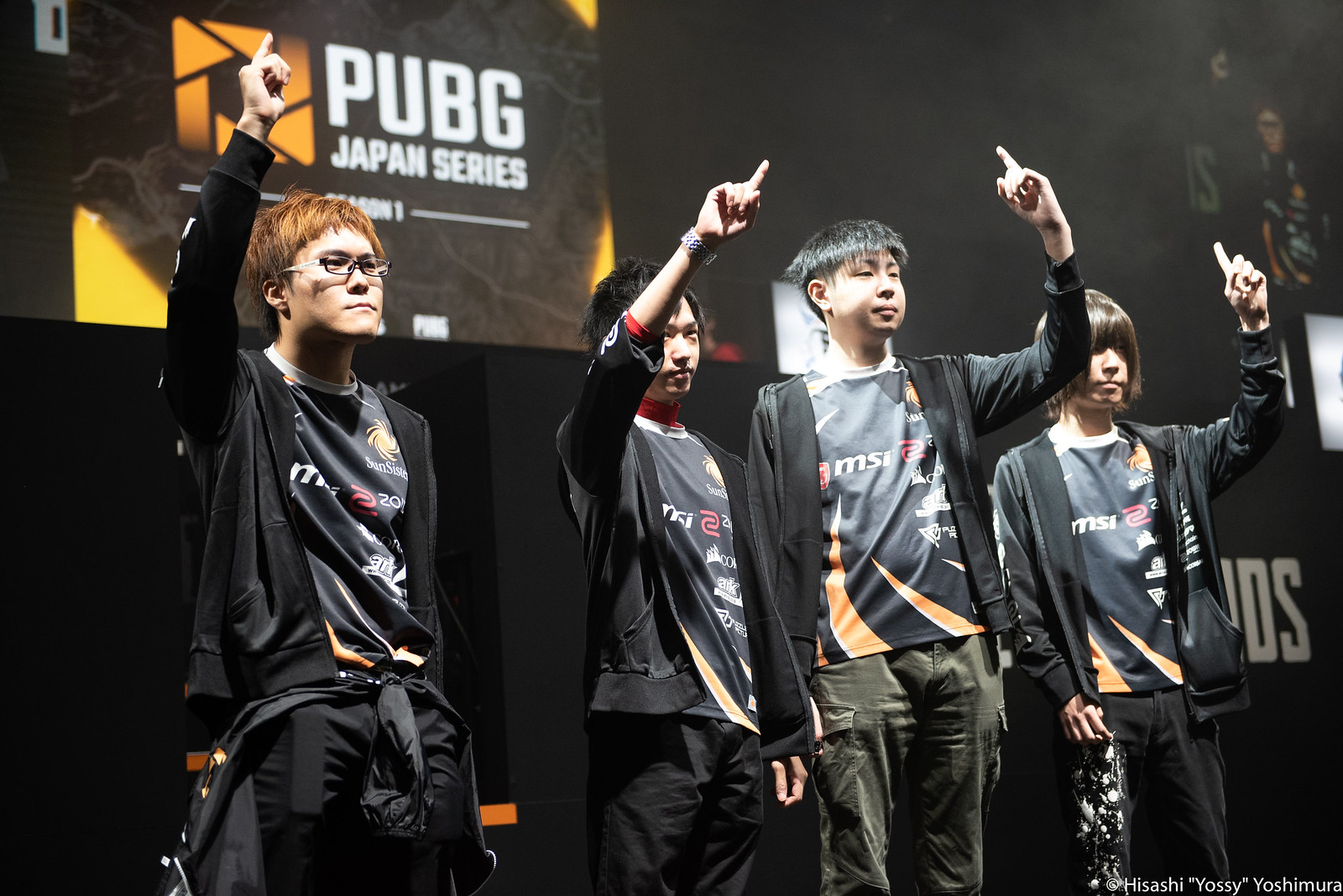In this detailed scene, four young Japanese men are standing on a stage, each holding their right hand up with the pointer finger extended, indicating the number one. They are all wearing black jackets over black or grey MSI jerseys, which feature a design resembling black and orange claws. Three of the men are dressed in black pants, while the second man from the right stands out with green camouflage pants. The man on the far left has red, short hair and wears glasses; the others have short black hair. In the bottom right corner of the image, the name Hisashi "Yoshi" Yoshimura is visible. Behind the men, a large projector screen displays the words "PUBG Japan Series" with dynamic black and yellow graphics. The men, who appear serious and focused, are standing in a line, looking in the same direction.